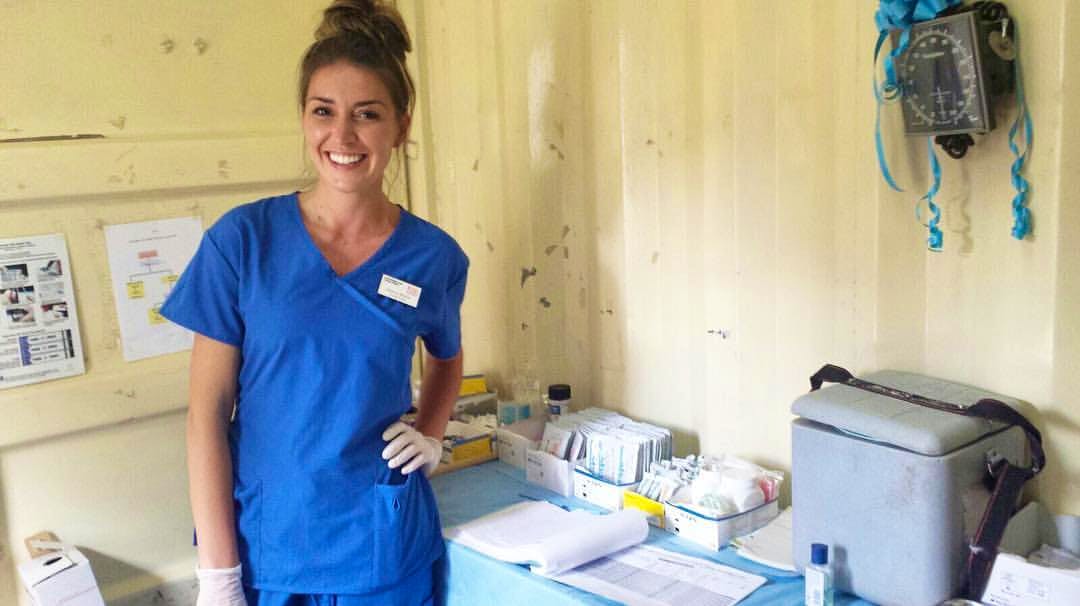A smiling brunette nurse stands confidently with her left hand on her hip, wearing blue traditional hospital scrubs and white nitrile gloves. Her name tag is attached to her left chest, and her hair is styled back in a bun with a few loose strands. She is photographed inside a mobile medical unit, indicated by the sheet metal, plastic-like ivory-colored walls, and the evident mobility of the space. 

In the background, a mix of medical equipment and supplies is visible: a blood pressure machine hangs on the upper right wall, various diagrams and charts are posted around, and a light blue tablecloth-covered table in the foreground is neatly arranged with medical tools, bandages, gauze, and possibly Germ-X. There's also an older-looking light gray cooler with a black strap, likely used for storing vials, suggesting this setup might be for vaccinations or blood draws. The overall scene is organized and professional, emphasizing the functionality and readiness of the mobile unit.